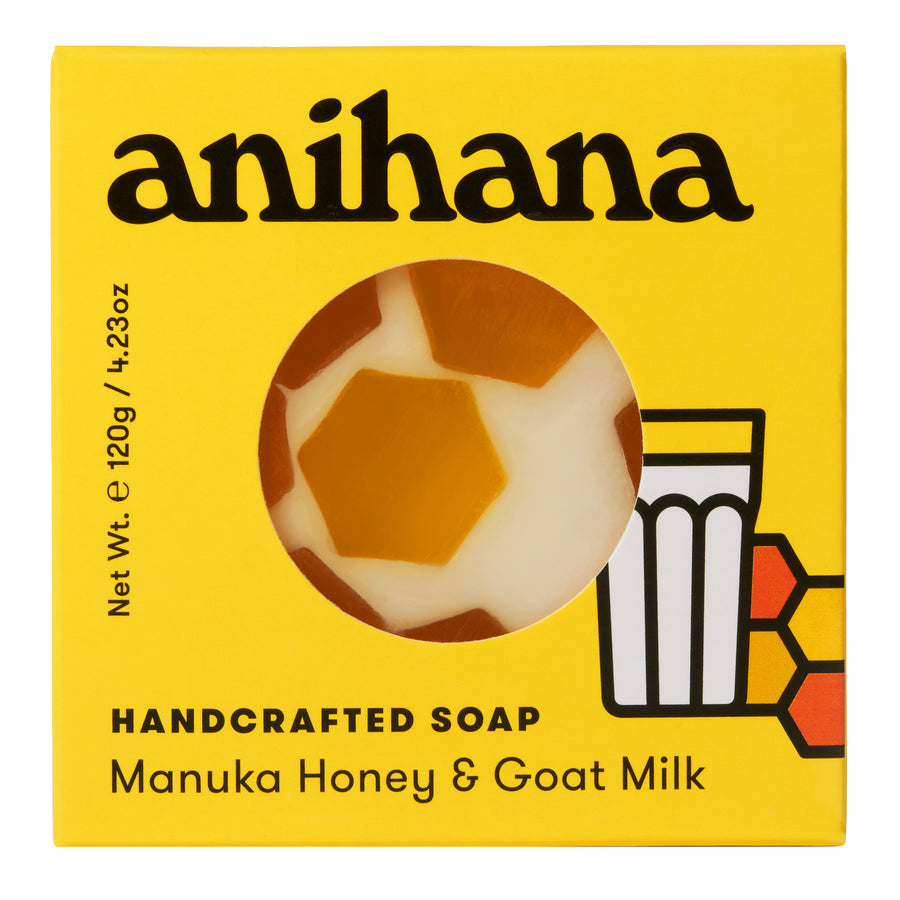The image features an advertisement for a brand of handcrafted soap named "Anahana." Dominating the background is a vibrant yellow color. At the top of the image, in bold, lowercase black letters, the brand name "anihana" is prominently displayed. Below this, a circular cut-out reveals the actual soap, which is intricately crafted to resemble a soccer ball, featuring six-sided shapes in brown and white hues, evoking the appearance of honeycomb.

To the right of this central circular section, there is a whimsical illustration of a nearly full glass of milk, outlined in black, accompanied by honeycomb shapes rendered in shades of orange and yellow with thick, bold outlines. Beneath the circular soap display, the label reads "Handcrafted Soap Manuka Honey and Goat Milk" in black font. Additionally, along the left edge of the image, in vertical text, the net weight of the soap is indicated: "120 grams / 4.23 ounces."